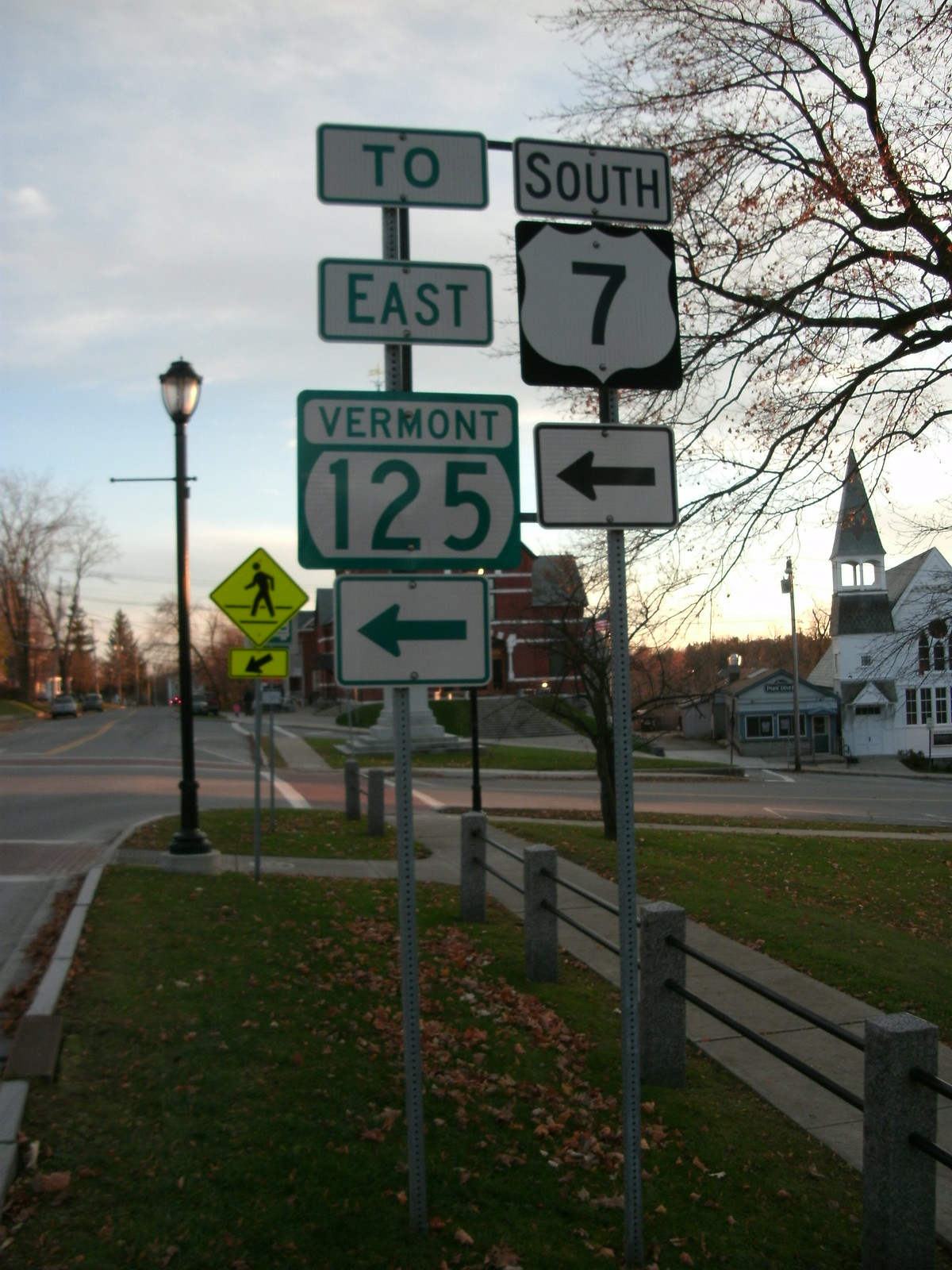A picturesque scene with late-autumn elements unfolds in this detailed image. The sky, a vibrant shade of blue with scattered clouds, serves as a backdrop to a number of dormant trees, their branches bare and devoid of leaves. Dominating the background is a stately church with white walls and a prominent bell tower topped with a cone-shaped roof. 

In the foreground, a street stretches on, its surface predominantly gray, reflecting a subtle glow from nearby streetlights. A yellow pedestrian crossing sign with a walking man illustration is visible near the corner of the street, adding a pop of color to the muted palette.

Additional street signage includes indications for Vermont Route 125 and directions for east and southbound travelers. Notably, above one of the signs, an airplane graphic can be spotted, hinting at a nearby airport or flight path. A charming lamppost, designed in a lantern style, further enriches this detailed and tranquil street scene.